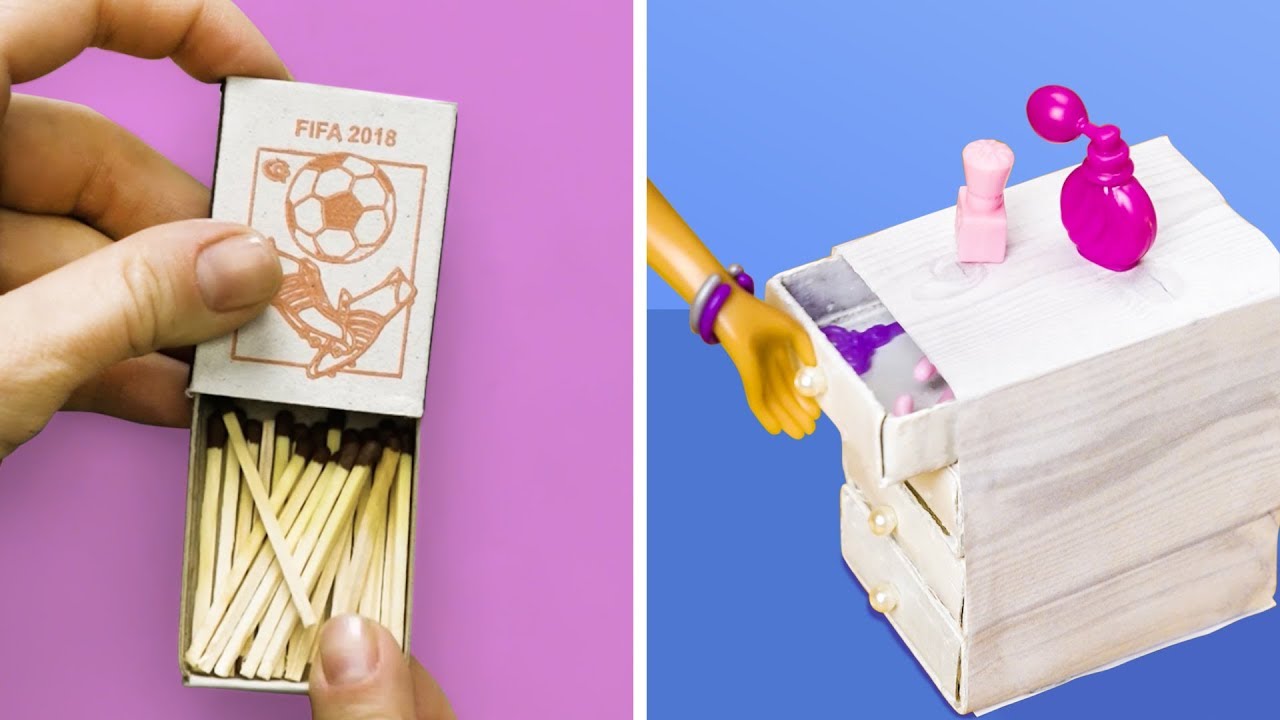The image consists of two distinct photographs side by side, both in vibrant colors. The square photograph on the left features a pepto-bismol pink background and shows a close-up of someone's hand holding and opening a traditional matchbox. The matchbox itself is white with a light brown logo that reads "FIFA 2018," accompanied by an illustration of a soccer ball and a pair of soccer cleats. The box has been slid open to reveal black-tipped matches inside.

The photograph on the right, with a blue background, depicts a Barbie doll hand, adorned with bangles, reaching down from below the elbow to open a tiny four-drawer dresser. On top of the dresser, there are small plastic accessories, including a pink perfume bottle and a lipstick. Inside the open top drawer, additional miniature doll accessories like an earring and a comb can be seen.